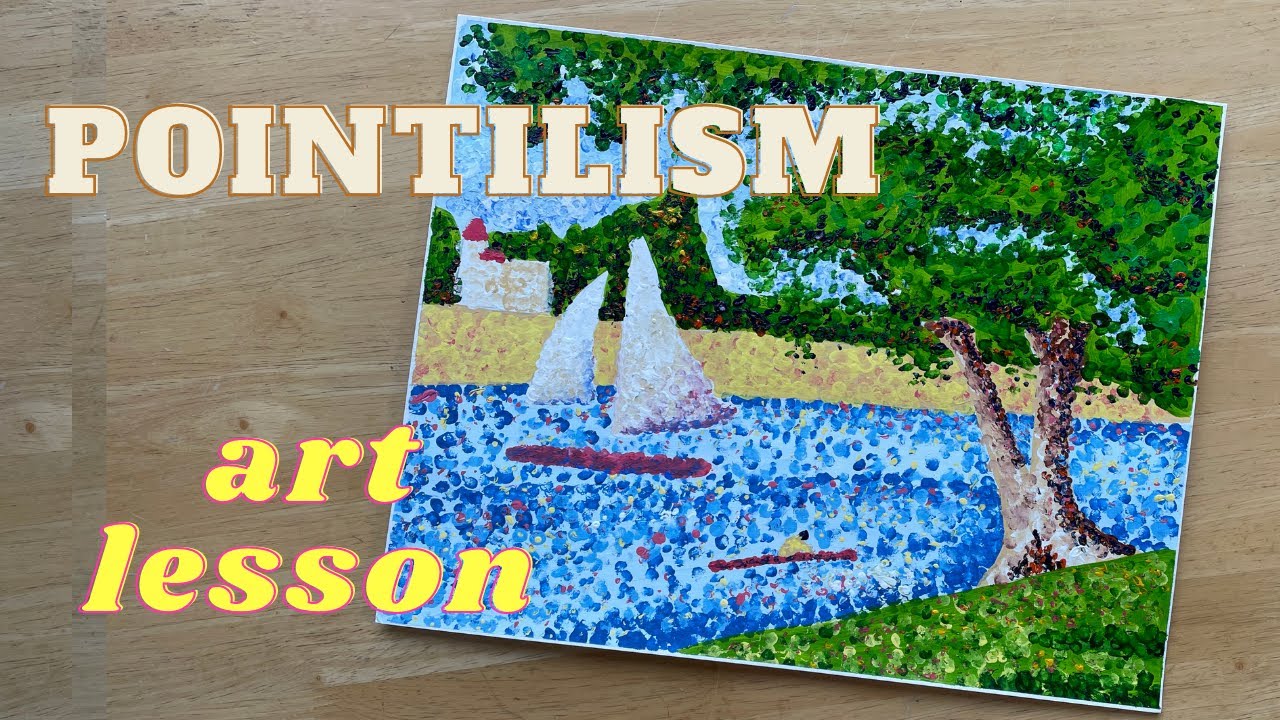The image appears to be an advertisement for art lessons focusing on pointillism. The background is a light brown wooden table surface. At the top left corner, the word "Pointillism" is written in beige letters, and below it, “Art Lesson” is written in yellow. Positioned at an angle on the right side of the table is a pointillist painting. The painting, created with numerous colorful dots, depicts an outdoor scene. In the foreground, there's a large brown tree with green leaves on a small hill, and a blue river with a boat on it. A person in a yellow shirt and black hair paddles a canoe on the river. In the background, there's a yellowish field, a beach, and a white house with a red roof. There's also a hint of hills or mountains in the distance.